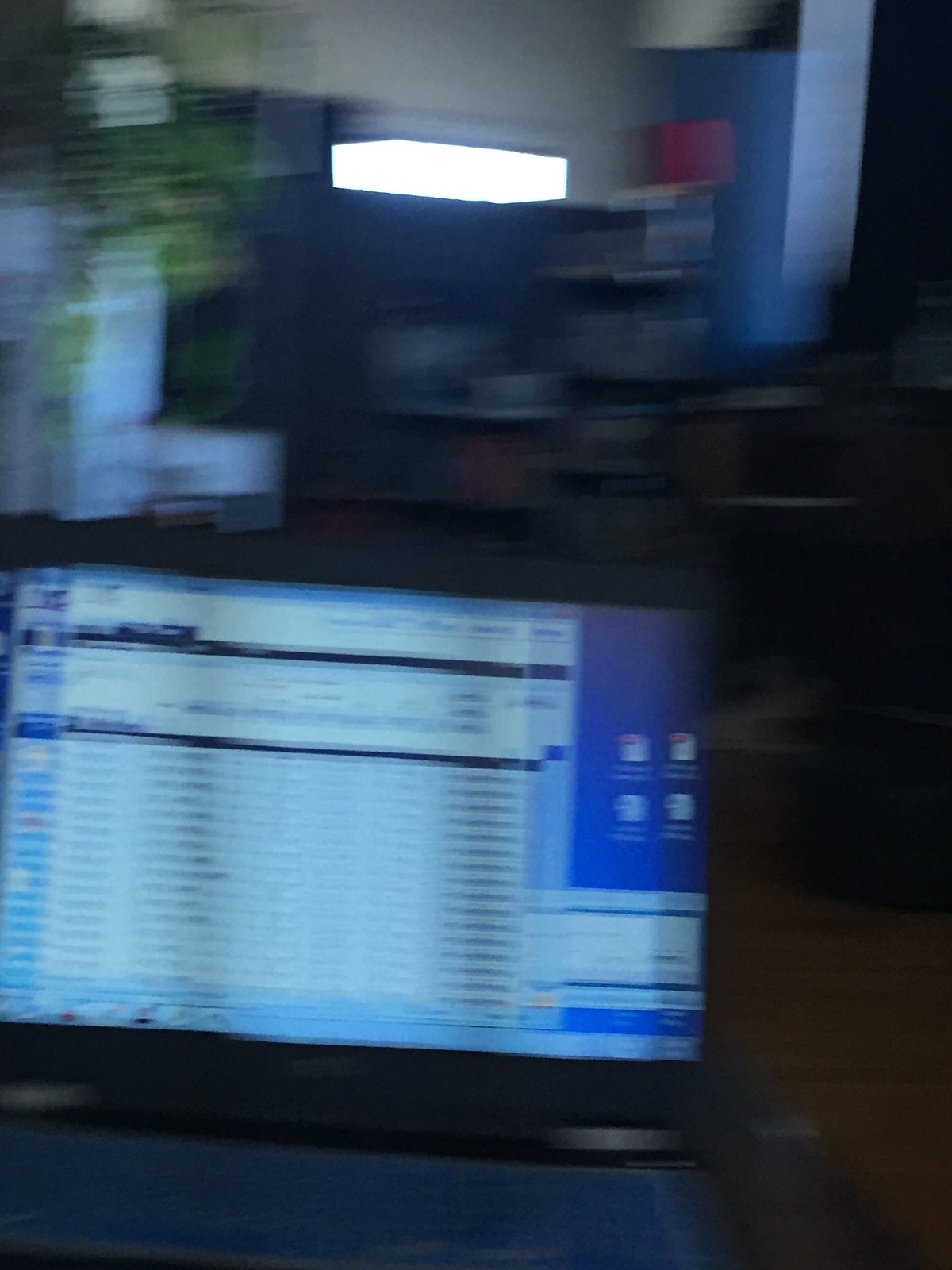This enigmatic image primarily features tones of blue and black, with a subtle illumination emanating from the upper portion. The overall composition lacks immediate clarity but invites deeper examination. Dominating the scene is a large dark blue square, punctuated by four smaller illuminated areas. This structure appears to be part of a dimly lit passageway flanked by indistinct buildings. Protruding from the top of the dark blue square are posts that resemble lampposts or streetlights, faintly suggesting an urban setting. On the right side of the image, a black shape with a prominent white slot is visible, possibly depicting an open doorway with a light source inside, adding to the mysterious ambiance of the photograph.